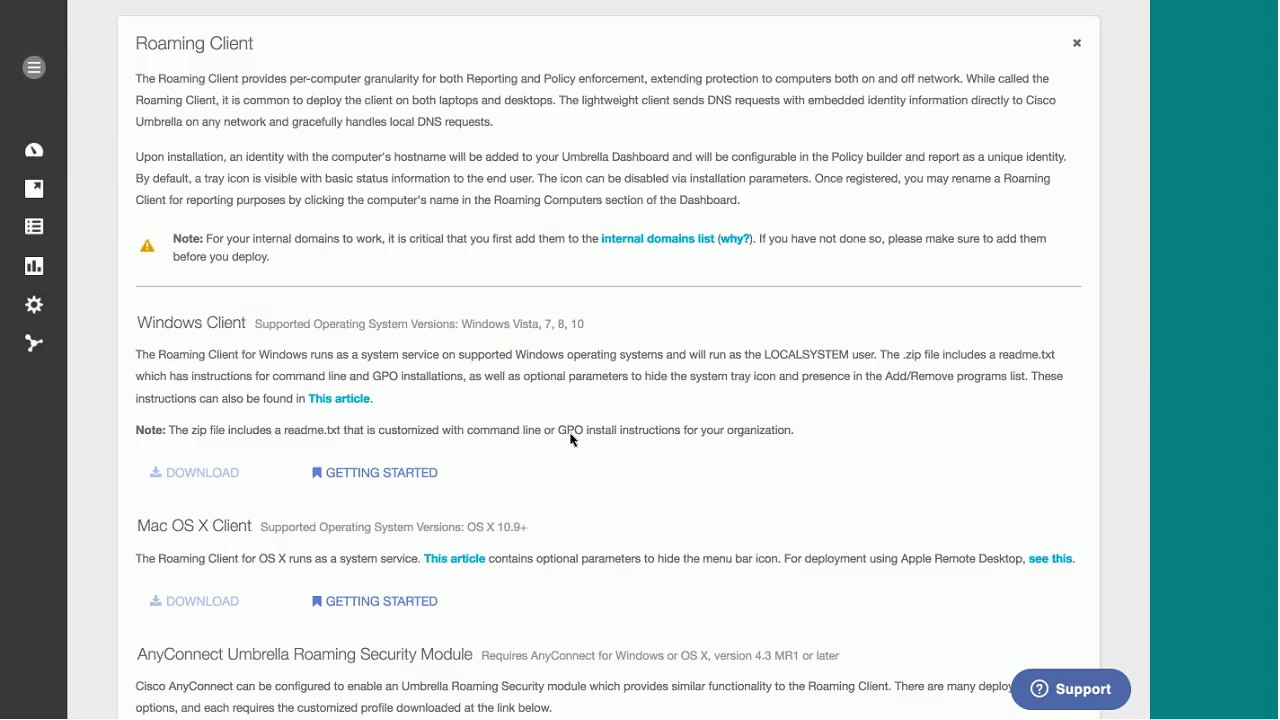This image is a detailed screenshot of a software application interface. On the left-hand side, there is a vertical, grayed-out navigation bar featuring six different icons from top to bottom: a cog wheel (settings), an arrow (navigation), a list, and a graph, among others. This bar also includes a section to expand and reveal additional options.

In the central portion of the image, a significant amount of text starts with a header titled "Roaming Client." This section describes the roaming client and includes a note that reads: "Note: For your internal domains to work, it is critical that you first add them to the internal domains list. If you have not done so, please make sure to add them before you deploy." Here, "internal domains list" and "add them" are highlighted in blue, indicating clickable links.

Below the roaming client information, there is another section titled "Windows Client" with additional text. This part includes a clickable link labeled "this article," also highlighted in blue. 

Below this information, there are two download buttons, one for Windows and one for Mac OS, displayed in light gray. Adjacent to these download buttons, two "Getting Started" buttons are visible in dark blue.

Further down, there's a section dedicated to the Mac OS X client, followed by a final section that discusses the "AnyConnect Umbrella Roaming Security Module," providing related information.

On the right-hand side of the image, a conspicuous support button is available for users seeking additional help.